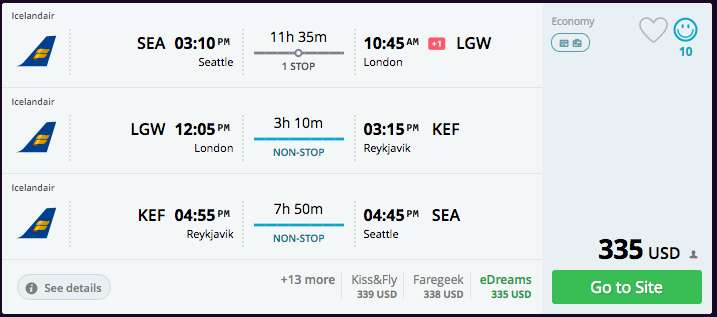This screenshot depicts a flight comparison website, showcasing travel options and prices for various flights. The featured flights are provided by Iceland Air, with the following routes and durations: an 11-hour and 35-minute flight from Seattle (SEA) to London Gatwick (LGW), a 3-hour and 10-minute flight from London Gatwick (LGW) to Keflavik (KEF), and a 7-hour and 50-minute flight from Keflavik (KEF) to Seattle (SEA). All flights are listed in the economy class.

At the bottom of the screen, several price options are displayed: Kiss and Fly at $339, FareGeek at $338, and eDreams at $335. The user has selected eDreams for its lowest price of $335, with an available button to proceed to their site. 

In the top right corner of the screenshot, there are interactive elements including a heart icon likely for saving favorites, and a smiley face with the number 10 underneath, which might represent user ratings or feedback. Additionally, the interface indicates 13 more pricing options that users can explore for further comparison.